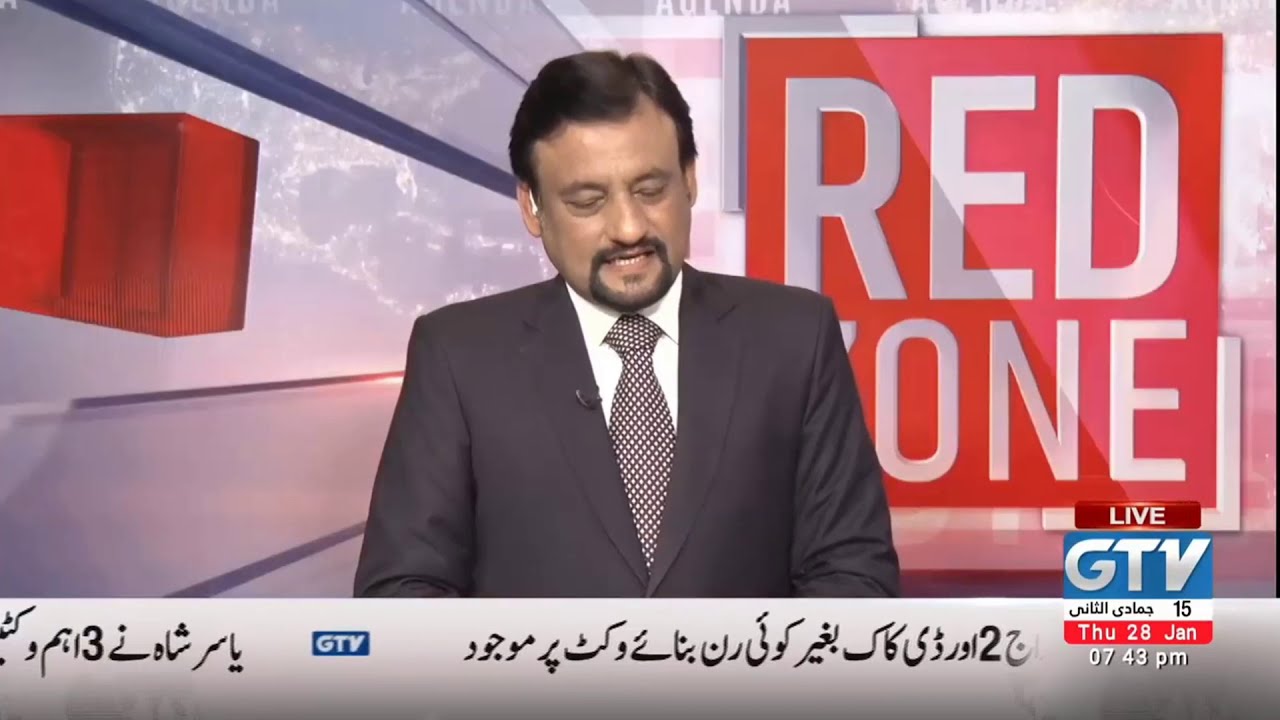The image depicts a still from an Arabic-speaking news program. The central figure is a middle-aged male newscaster with brownish skin, black hair gently parted to his left (our right), and a distinct facial appearance featuring a black mustache and a small beard limited to his chin. He is dressed in a gray suit, a gray polka-dotted tie, and a white shirt, with a small microphone clipped to his lapel and a white earpiece in his right ear (our left). He is looking slightly downward, appearing to read something with his mouth slightly open, revealing his bottom teeth.

In the background, on the right side of the screen, there is a large red square with the text "Red Zone" in silver or gray lettering. Below this, in a red block with white lettering, it says "Live." Further down, in a blue block with white lettering, it displays "GTV." Beneath this, there's additional script in Arabic, accompanied by the number "15" in black. Directly beneath, another red block shows "THU 28 JAN," and the time "07:43 PM" is displayed below. The scene is accentuated with futuristic graphics, including the shape of a globe and dynamic lines in blue and red tones. Additionally, a white banner with black Arabic text, interspersed with blue rectangles containing the letters "GTV," runs along the bottom of the screen.